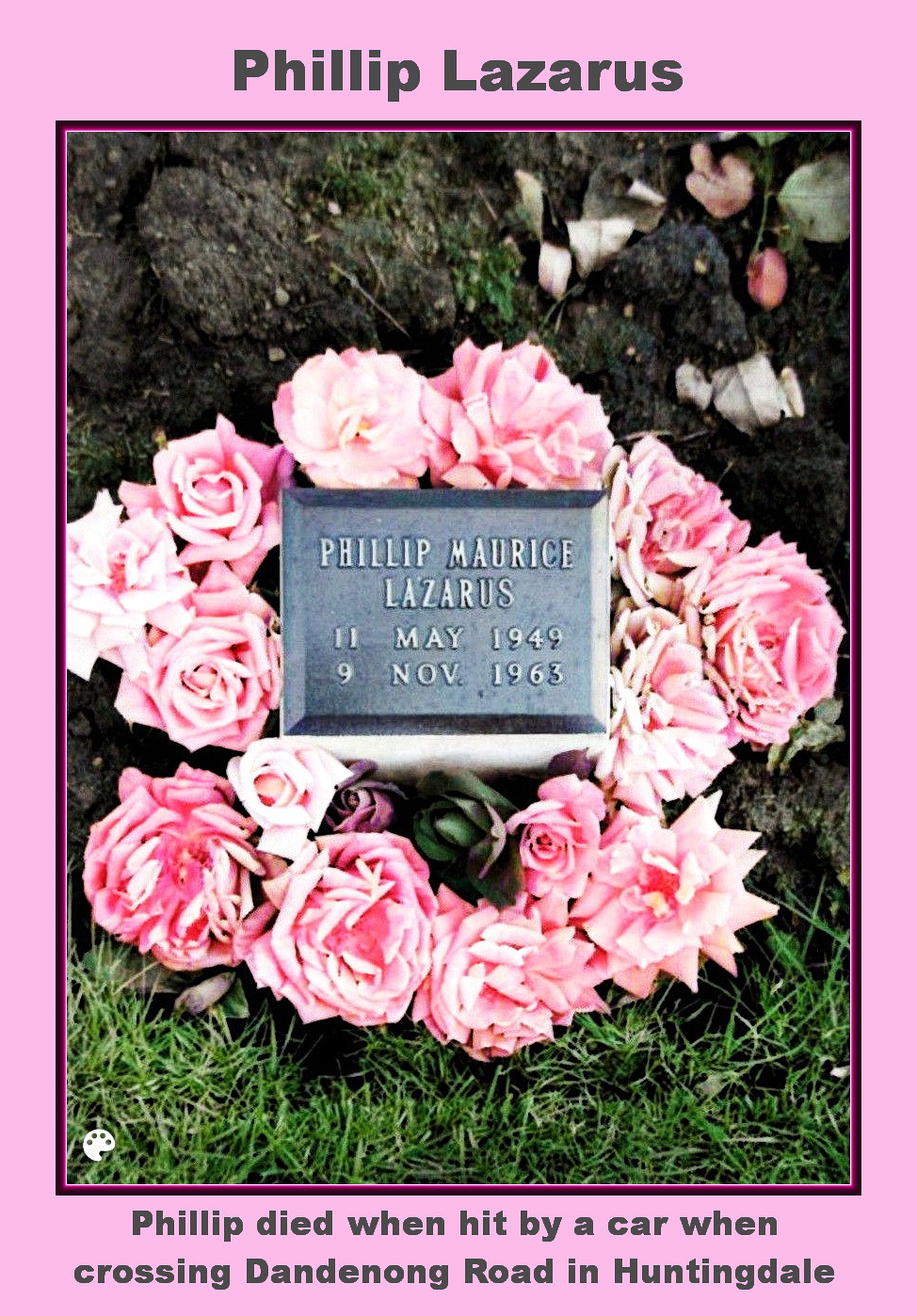The photograph depicts a somber scene bordered by a pink frame, focusing on a small gravestone nestled within a ring of pink flowers. The gravestone, made of metal with edges cut to show varying depths, features raised lettering. It reads "Philip Maurice Lazarus" on the first line and "Lazarus" on the second line. Further details inscribed include "11 May 1949" and "9 November 1963," indicating the lifespan of the deceased. The background includes rocks and patches of grass, suggesting a natural setting. At the top of the image, within the pink border, it states in gray text, "Philip Lazarus." At the bottom, also in gray text, it is noted that "Philip died when hit by a car when crossing Dandenong Road in Huntingdale."